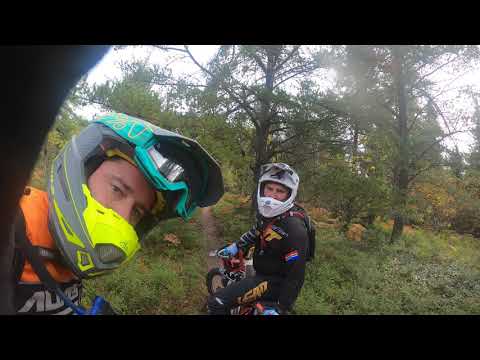A vibrant selfie captures two young, light-skinned men gearing up for a mountain bike adventure through a lush forest. The photo is framed with a dark black border on the top and bottom, emphasizing the richness of the scene. The man on the left, who holds the camera, stands out in his orange and black jersey adorned with white text, and a grey helmet with neon yellow highlights. His blue-rimmed goggles rest firmly over his eyes. To his right, a companion is poised on a red and black mountain bike. This second biker is clad in black pants, a black jacket, and blue gloves, with white-rimmed goggles perched atop his white helmet. They sit on a narrow dirt path, surrounded by tall green grass and trees bursting with green leaves. The forest background adds a sense of adventure and tranquility, punctuated by the bright, cloudless white sky peeking through the dense tree canopy.